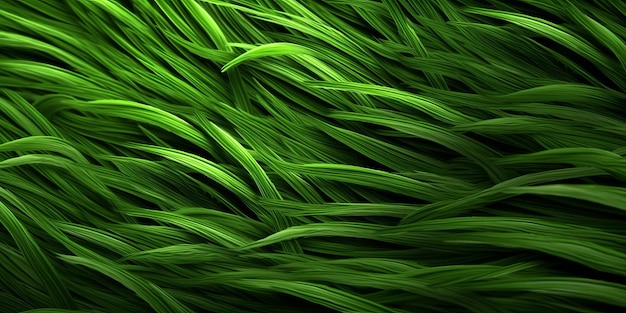The image showcases a detailed close-up texture in varying shades of green, reminiscent of feathers or blades of grass. The elements appear uniformly shaped and curve uniformly in the same direction. They are layered on top of each other, creating an intricate, almost braided appearance. The composition features a gradient of light, with the upper left-hand corner brightly illuminated, casting a luminous glow on some areas, and progressively darkens towards the bottom and right-hand side. The visual texture is mesmerizingly abstract, inviting interpretations that range from shaggy bird feathers to large, overlapping leaves or even a microfiber material, owing to its finely detailed and layered presentation.